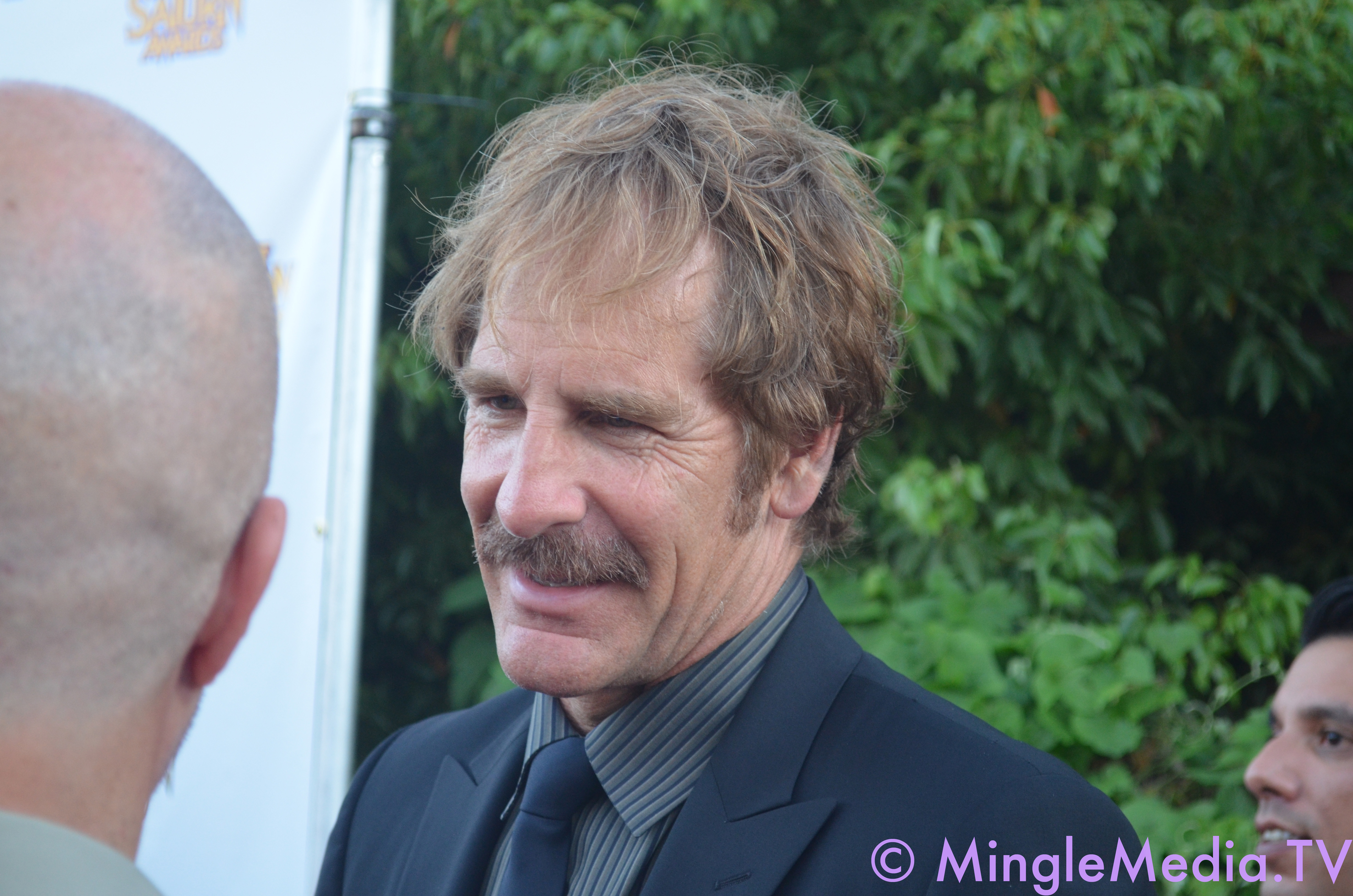The photograph features a man centered in the frame, facing slightly towards the bottom left. He is dressed in a dark blue business coat over a grey button-up shirt with blue stripes and a matching blue tie. The man has an unkempt blonde mustache tinged with specks of grey and medium-length, slightly messy blonde hair. His image is cut off at the chest.

In the background, there is tall greenery, possibly trees or bushes, creating a natural setting. To the left edge of the photograph, a portion of a bald man's head with dark spots where hair might grow is visible, showing just his right ear and part of his shirt collar. This man appears to be who the central figure is addressing or looking at.

Additionally, in the bottom right corner, the face of another man looking to the left is partially visible, cut off by the edge of the photo. A purple watermark reading "© Mingomedia.tv" is present in this corner as well. Both captions suggest that the central figure in the image might be Scott Bakula.